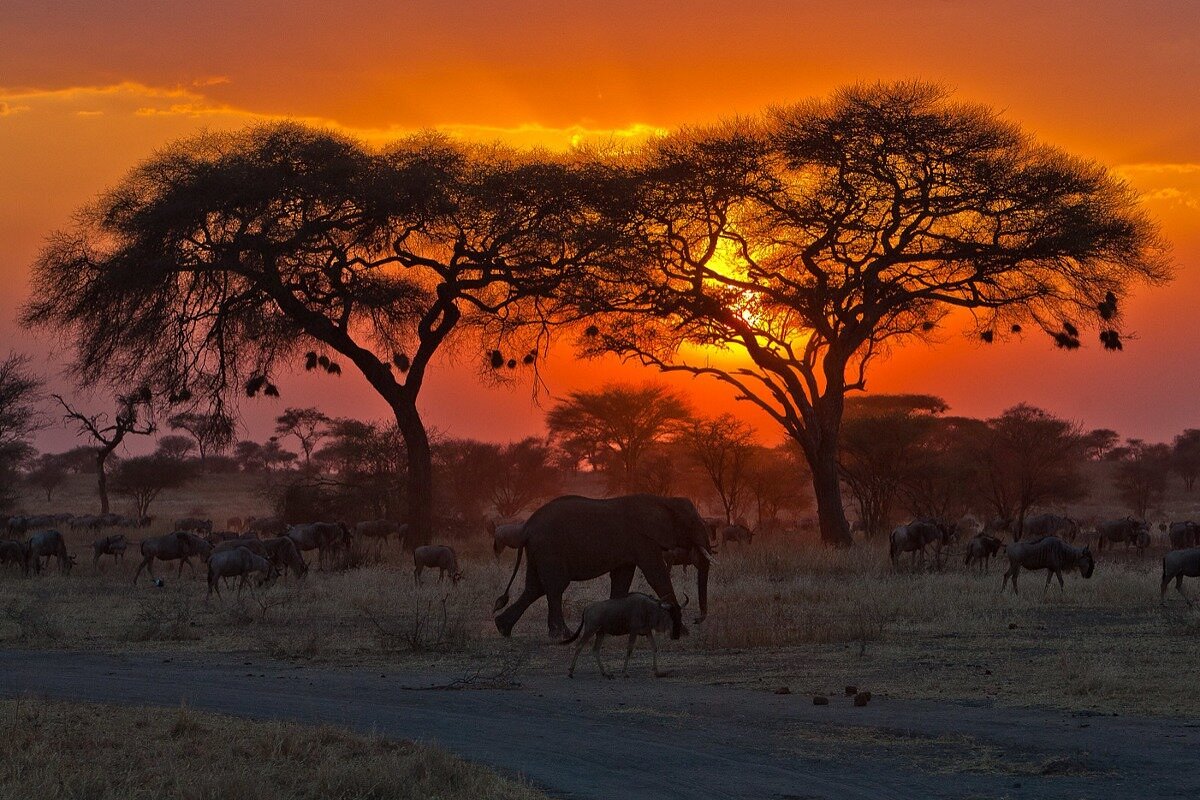This photograph captures the serene beauty of a savannah, likely in Africa, during either sunrise or sunset. The sky, bathed in a gradient of red to vivid orange, forms a striking backdrop. In the foreground, the silhouette of a majestic elephant is prominently visible, accompanied by several smaller animals, likely antelopes. They traverse a barren landscape with sparse, brown, and dried-out grass, possibly indicative of winter or a dry season. A discernible road cuts through the plain, hinting at a safari route in this peaceful, rural setting.

Two distinct trees stand against the illuminated sky, their bent trunks and branches reaching leftward. These trees are sparsely foliaged, allowing glimpses of the colorful sky through their leaves. Additional, more distant tree silhouettes pepper the horizon, enhancing the depth of the scene. The overall image strikingly juxtaposes the dark, detailed foreground against the bright, glowing sky, encapsulating a moment of tranquil natural splendor.